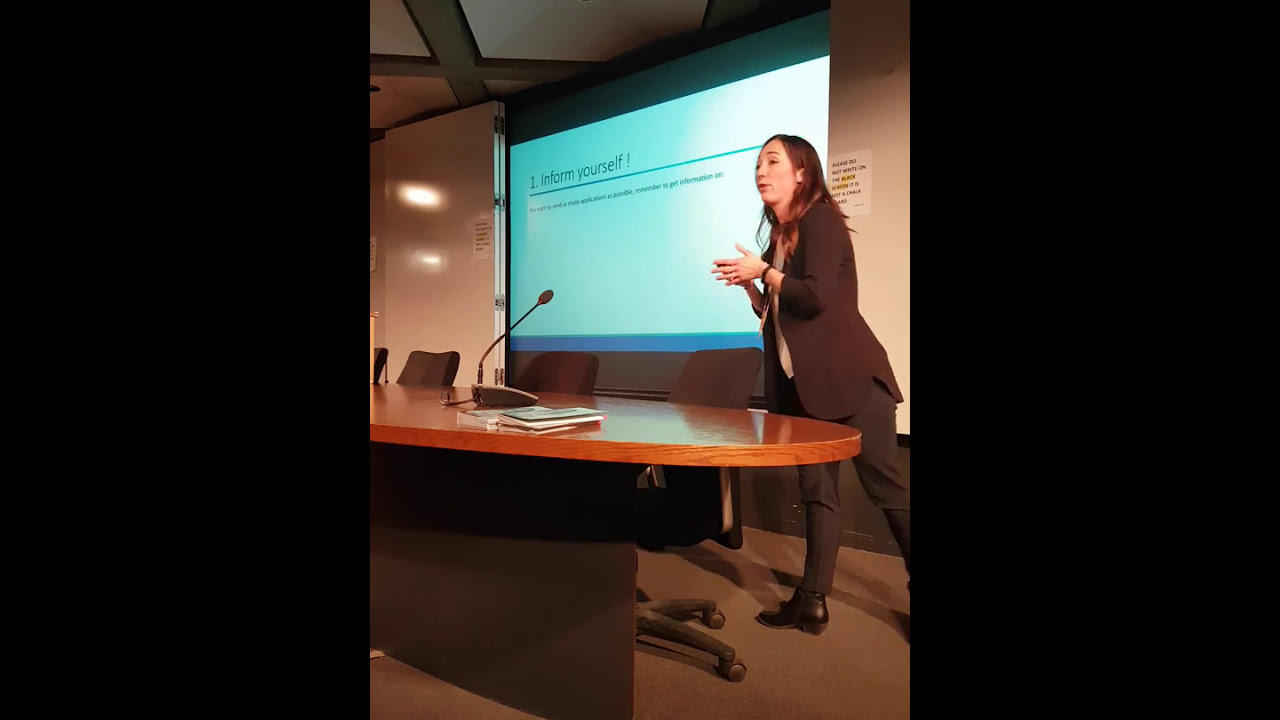In the image, a woman with light skin and shoulder-length brown hair, wearing a brown suit with brown pants and a cream-colored shirt, is standing in a well-appointed meeting room. She has a black watch on her wrist and a bracelet, and her hands are held up in front of her chest. One foot is flat on the ground while the other is extended behind her, poised on her toes. She appears to be giving a presentation, standing behind a long oval wooden table surrounded by cushioned brown office chairs on wheels. In front of her on the table is a microphone and what appears to be a telephone.

Behind her, there is a large dropped-down screen with a teal background displaying the text "Inform yourself!" along with additional, unreadable text below a blue line. The screen is likely part of a projector setup. The room has a white wall, a door visible to the left, and a ceiling with a grid-like pattern in white, gray, and brown hues. A barrier panel runs along the front of the table, concealing the underside where people’s legs would be when seated. Sunlight or another light source casts a glare on the wall to the left, contributing to the well-lit ambiance of the space. Various papers, some highlighted, are also on the table, indicating a detailed and informative presentation setting.